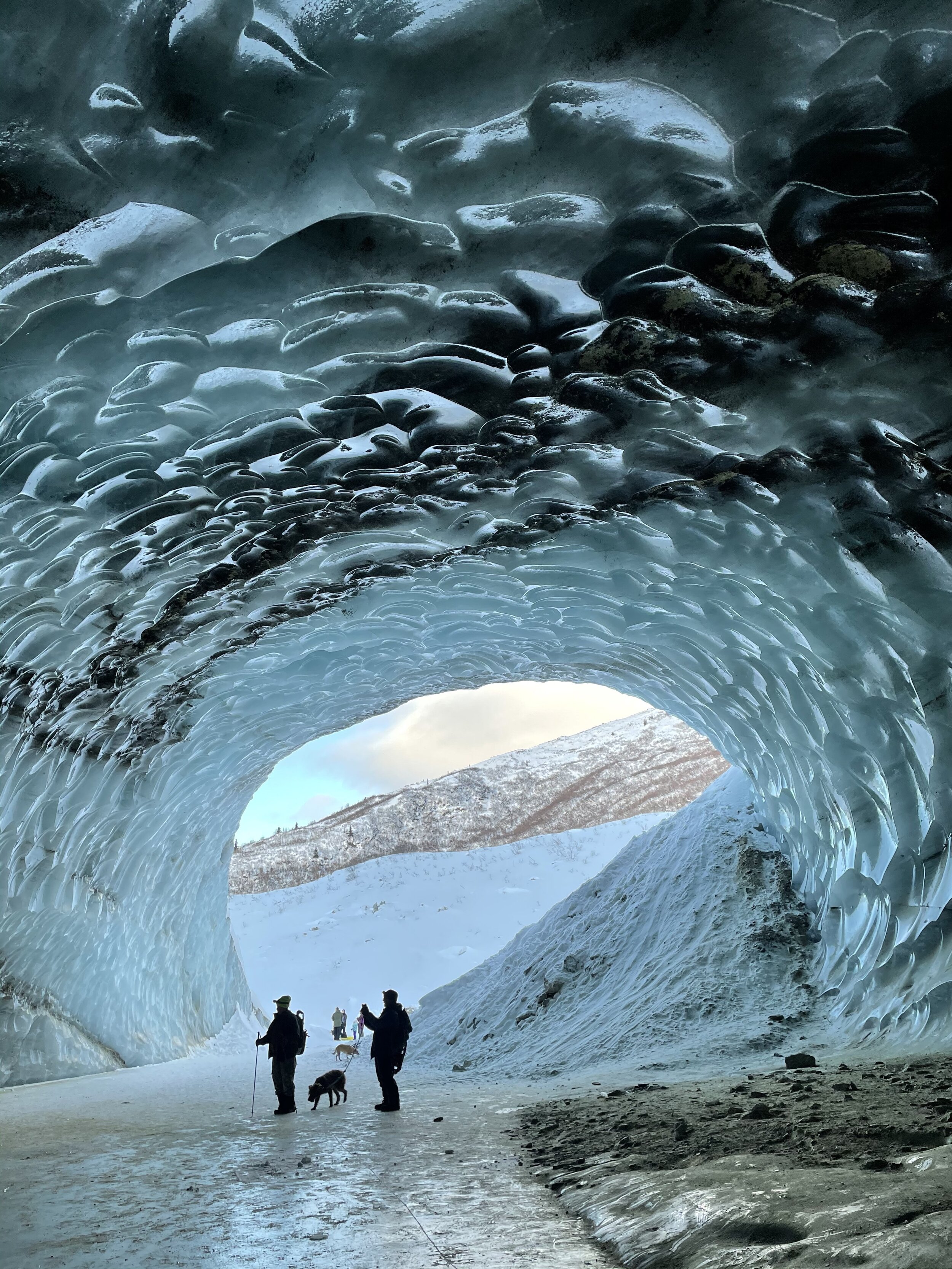The photograph captures a stunning scene of a frozen ocean wave, which has formed a tunnel large enough to walk through, resembling an ice cave. The tunnel, with its black and white ice ceiling bearing grooves formed by melting and refreezing, creates an almost surreal passageway. The ground inside the cave is a mix of slippery ice, dirt, rocks, and patches of mud and water. Several warmly dressed people, some using hiking sticks, are exploring the icy path, accompanied by two dogs. The sun illuminates the scene and a clear blue sky stretches above, framing a distant, snow-covered mountain with dark grey patches. The scale of the tunnel makes the people appear small, highlighting the immense size of this natural ice formation.